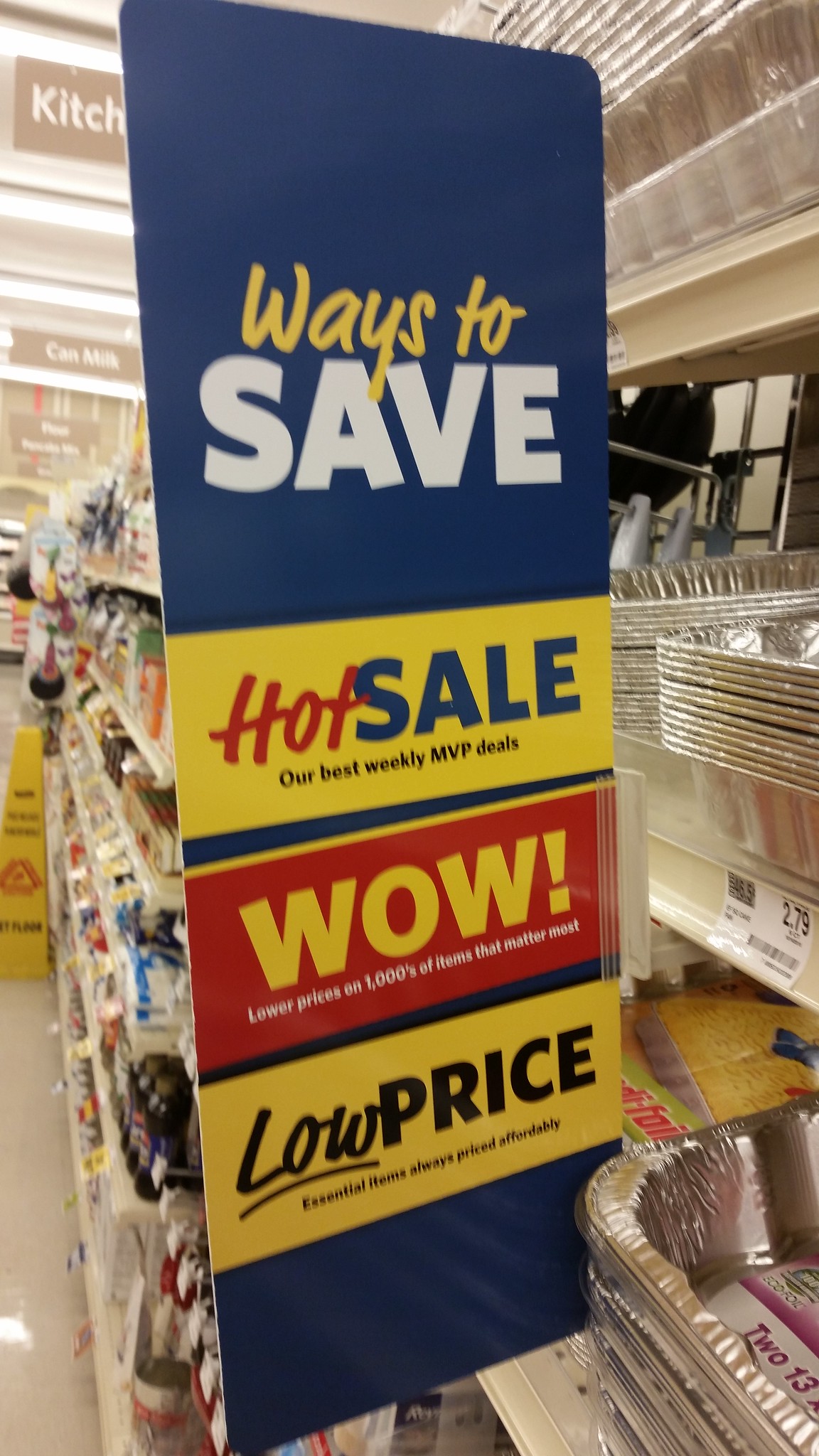The photograph captures an aisle inside a grocery store, likely a Walmart, featuring metal beige shelves on the right. In the center-right of the image, a prominent rectangular sign, primarily in blue, yellow, and red, draws attention. The sign is divided into multiple sections: 

- The top section is blue and reads "WAYS TO SAVE," with "save" in large white capital letters and "WAYS TO" in yellow.
- The next section is yellow, displaying "HOT SALE," with "HOT" in red and "SALE" in blue.
- Below, a blue stripe states "OUR BEST WEEKLY MVP DEALS."
- Further down, a red stripe exclaims "WOW!" in large yellow capital letters.
- Underneath, the message "lower prices on thousands of items that matter most" is written in white.
- The bottom section is yellow again, featuring "LOW PRICE," with "LOW" in an underlined cursive script and "PRICE" in capital letters.

Adjacent to the sign, metal shelves hold various kitchen utensils, including foil baking trays. Off to the left, a thin strip of beige linoleum or tile flooring is visible, with a yellow caution stand situated centrally on this side.